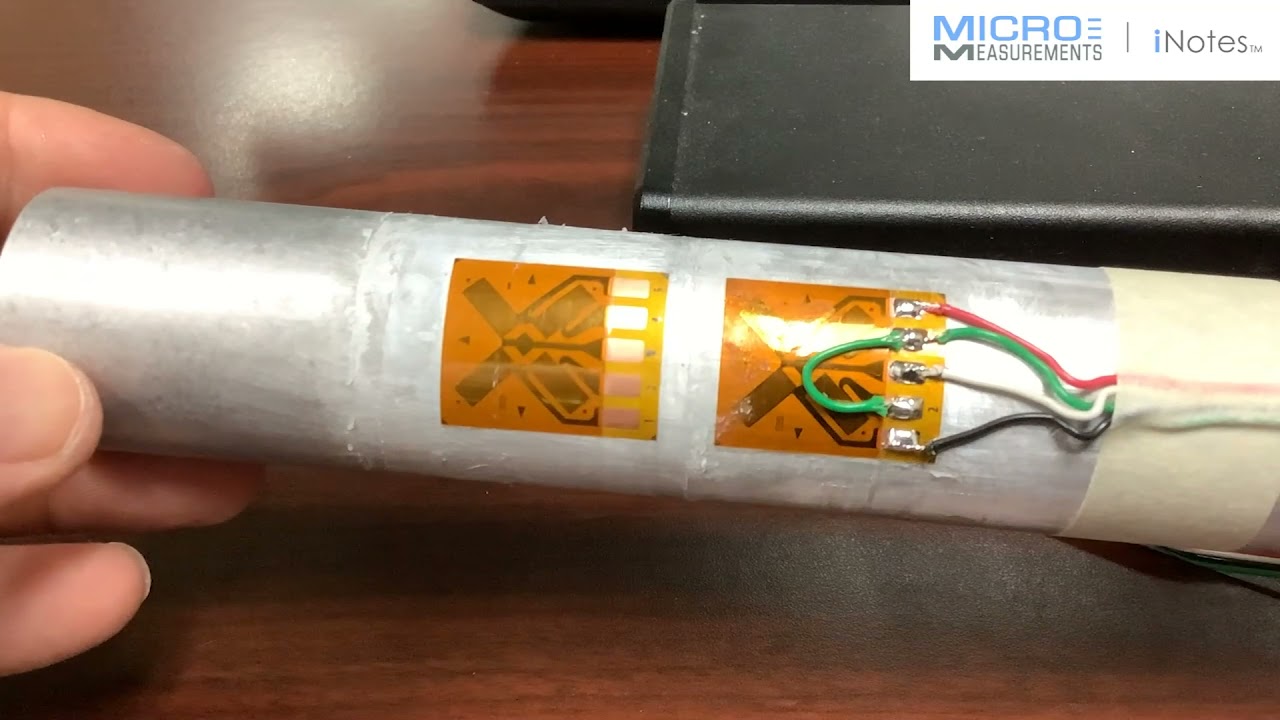The photograph captures a close-up of a rectangular metallic cylinder, silver in color, situated horizontally on a wooden desk surface. The cylinder has orange adhesive patches arranged vertically, one above the other, attached to its surface. The lower patch has wires soldered to it, secured with masking tape, featuring a red wire at the top, followed by green, white, and black wires. The top of the device is being lifted by fingers likely belonging to a white person's hand, barely visible on the left side of the frame. In the background, a black object, possibly a laptop, is partially visible. In the upper right corner of the image, the logo "Micro Measurements" appears, with "Micro" in blue font and "Measurements" in dark gray, followed by "iNotes" in the same dark gray font with the initial "i" in blue. A small trademark symbol is located at the lower right of the logo.